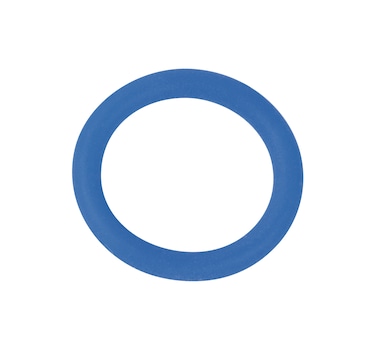The image features a minimalistic and sparse composition with a stark white background. Dominating the scene is a slightly lighter than slate blue circle, which sits prominently in the center. The circle, with a matte and flat finish, appears somewhat irregular and slightly oval rather than perfectly round. This blue hue is devoid of any highlights or lowlights, maintaining a consistent flat appearance.

The outer ring of the circle is of moderate to thick line width, reminiscent of a bold font, and could potentially be interpreted as the letter "O". The blue ring encompasses a pure white interior that echoes the background, giving the impression of a hollow circle or ring. Some portions of the blue outline exhibit lighter sections, creating an uneven and non-continuous effect, with variations in thickness suggesting a possible 3D effect or inconsistency in the ring's design.

This simple and abstract image, with its distinctive and straightforward visual representation, could easily find its place in educational materials such as math or children's books illustrating basic shapes and sizes.